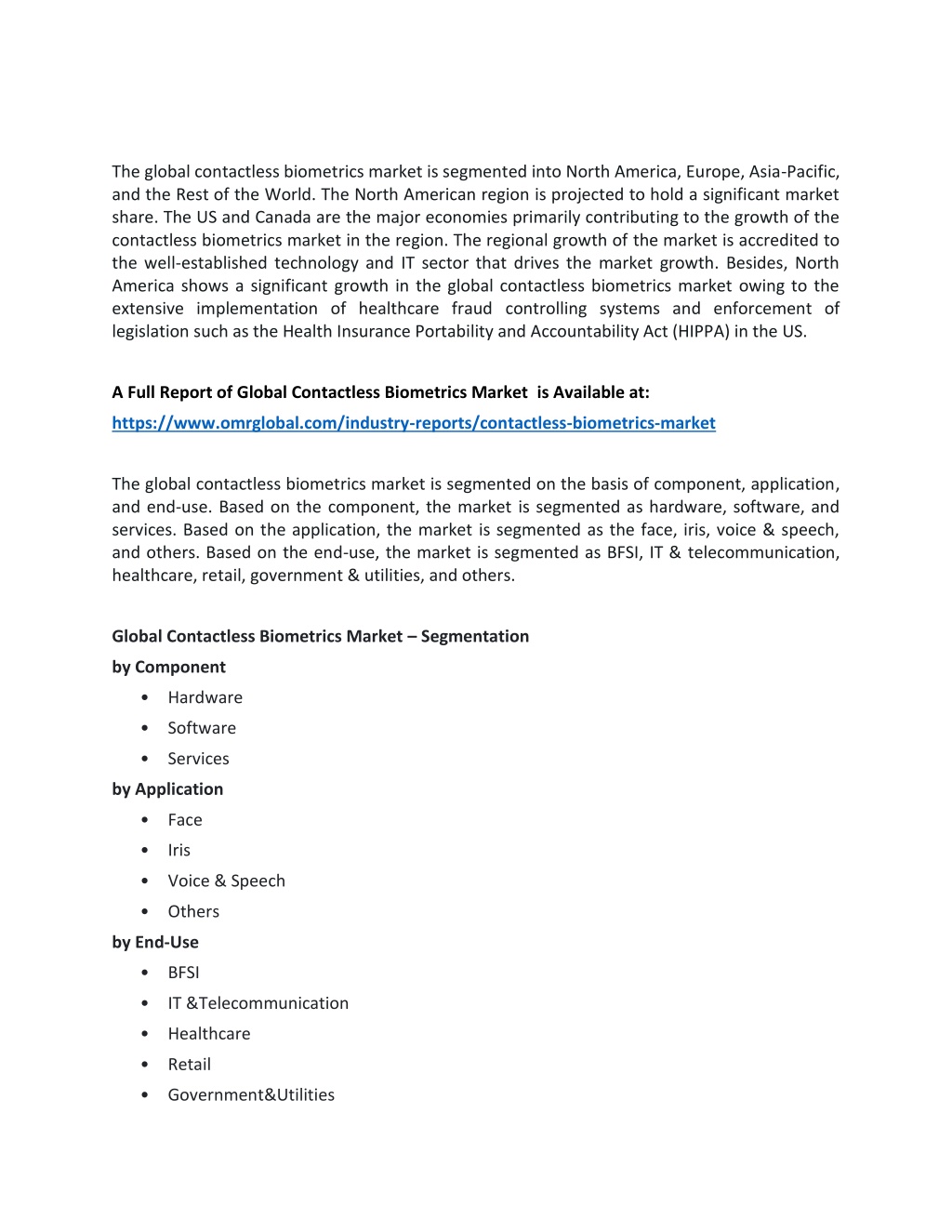The image features a detailed document or website page containing typed information, including a hyperlink. At the top, the text highlights the segmentation of the global contactless biometrics market, divided into North America, Europe, Asia-Pacific, and the rest of the world. 

North America is set to hold a significant market share, with the U.S. and Canada being the primary contributors to market growth. The region's growth is attributed to its advanced technology and IT sectors. Additionally, North America's implementation of healthcare fraud control systems and legislation such as the Health Insurance Portability and Accountability Act (HIPAA) in the U.S. further drive market expansion.

Readers are encouraged to view the full report on the global contactless biometrics market by visiting www.omrglobal.com/industry-reports/contactless-biometric-market.

The document further details that the global market is segmented by components (hardware, software, and services), applications (face, iris, voice and speech, and others), and end-use sectors (BFSI, IT and telecommunications, healthcare, retail, government and utilities, and others). Below this, the segmentation is reiterated, emphasizing the categorization by components, applications, and end-use sectors.